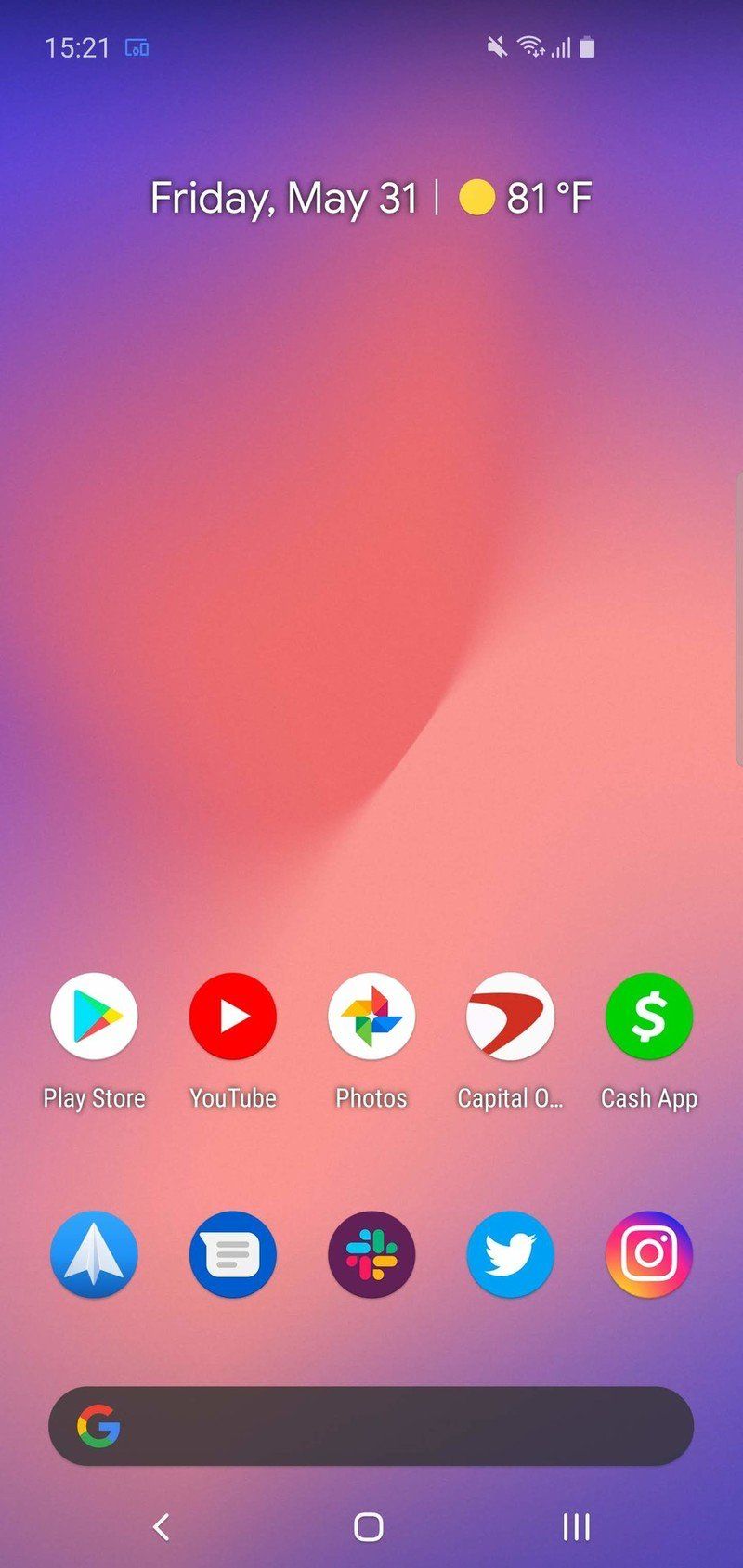The image depicts a cell phone screen with a vibrant and colorful background. The top section of the screen is adorned with a rich purple hue, transitioning to an orangey-red tone in the middle, surrounded by a peach-colored gradient, and returning to purple at the bottom. In the upper left corner, the time is displayed as 15:21. A blue notification box is also present.

On the right side of the screen, near the top, are several status icons indicating connectivity and battery life. The date is stated as "Friday, May 31st." Dominating the center of the image is a large yellow sun icon with a temperature reading of "81 degrees Fahrenheit."

The lower portion of the screen displays several app icons including "Play Store," "YouTube," "Photos," "Capital One" (indicated by a capital 'O'), and "Cash App." Additionally, there are notifications present, including a message notification with a brown icon featuring red, yellow, green, and blue lines radiating from its center, along with "Twitter" and "Instagram" icons.

Beneath the apps is a black search bar, featuring the Google 'G' logo on the left side. At the bottom of the screen are essential navigation icons: a phone icon on the left, a square in the middle, an arrow on the left, and three vertical lines on the right.